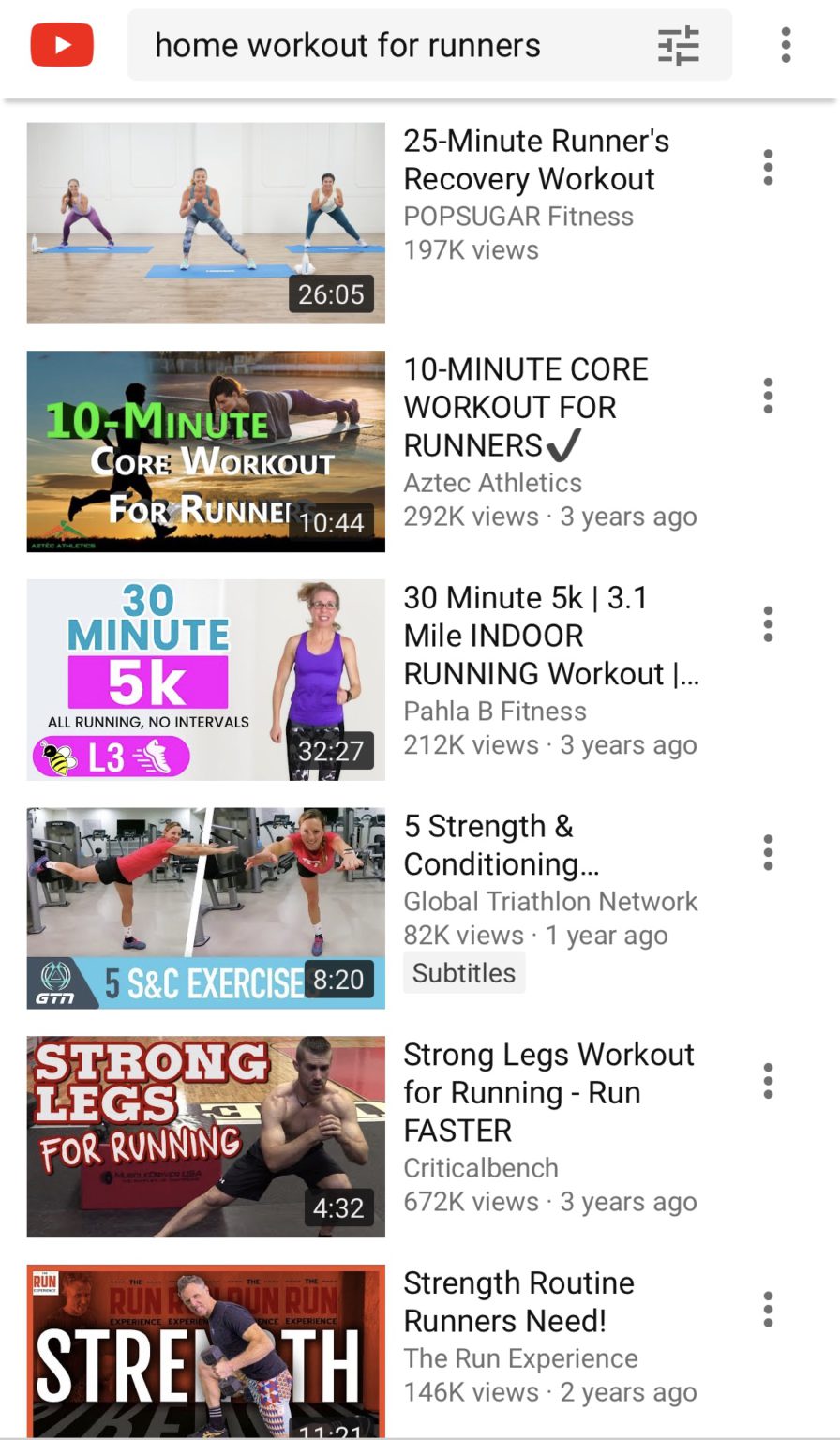The image depicts the YouTube app interface in light mode, characterized by a predominantly white background. The text input boxes are gray, while black accents are used for text and the three-dot menu buttons beside each video. At the top of the screen, there is a search banner where the user has entered "home workout for runners." To the left of the search bar is the YouTube logo, represented by an orange square with a white play button in the center.

Below the search bar, there are six videos related to the search term. The first video is titled "25-minute Runners Recovery Workout" and features a simple thumbnail with three people in a spacious gym area, standing on blue mats, dressed in tight exercise gear, and engaging in various workout activities. The second video, titled "10-minute Core Workout for Runners," has a prominent check mark next to the title and features a thumbnail with bold text.

Other videos include:
1. "30-minute 5K," featuring a colorful thumbnail with a pink backdrop behind the "5K" text.
2. "Strength Routine Runners Need," which has a thumbnail showing a man in front of the word "Strength."

Each video thumbnail follows the typical YouTube design, with some incorporating vibrant colors and large text to grab viewers' attention. The interface also shows clickable slider icons for advanced search options.